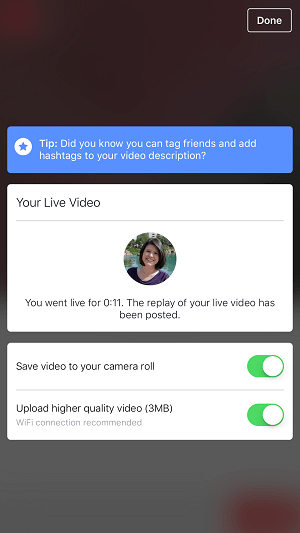"On the screen, there is a blue rectangle with a star icon indicating an option to tag friends and add hashtags to your video description. A white square displays the message 'Your Live Video,' showing a person with short hair with a blue wire background. It notes that the live video lasted 11 seconds, confirmed by the message 'You went live for 11 seconds' and 'The player live has been posted.' Another message prompts to 'Save video to your camera roll,' featuring a green oval toggle with a white circle inside. There is also an option to 'Upload higher quality video (3 MB, WiFi connection recommended).' The background is dark and slightly blurry towards the bottom, with a dark spot at the bottom right corner. In the background, pixelated text mentions a woman with very short black hair, contributing to the overall scene with its gritty detail."